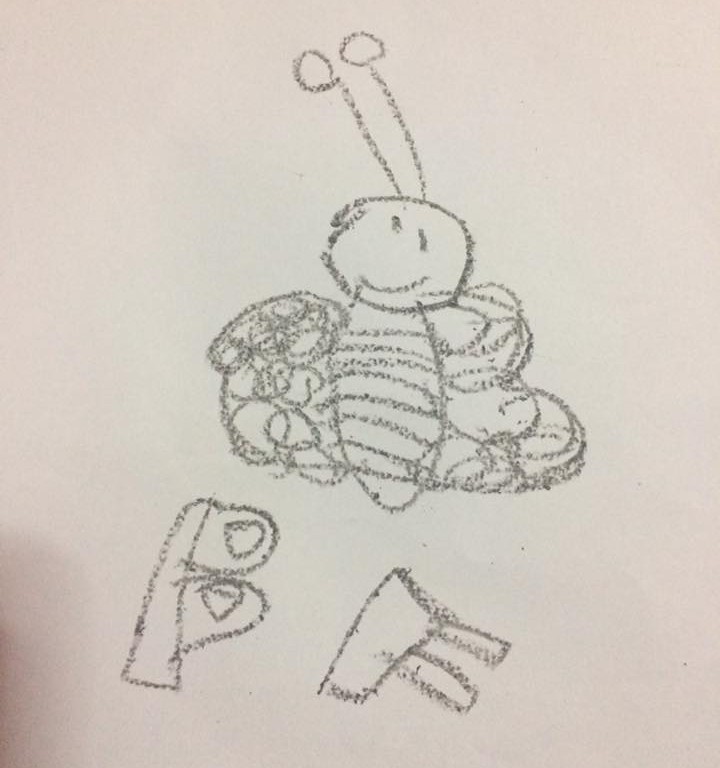The image depicts a rudimentary, black-and-white drawing that appears to be the work of a child. Dominating the composition is a large, circular-headed figure that resembles a butterfly or a bumblebee, drawn likely with a black crayon or marker. The head is accentuated with human-like features, including two eyes and a smiling mouth. Two long antennae, tipped with circles, extend from the head, enhancing its insect-like appearance. The body is an oval shape adorned with horizontal stripes, signifying a bee's characteristic markings. Fluffy, cloud-like figures on either side of the body represent scribbled wings. 

Below this main figure are two objects, perceived as bubble letters "B" and "F" with a small heart nearby, suggesting someone’s initials. The entire drawing rests on a white background, which lacks any visible edges, giving it a floating appearance. A small shadow can be seen to the left of the image, possibly indicating the drawing's texture or the lighting at the time it was photographed.